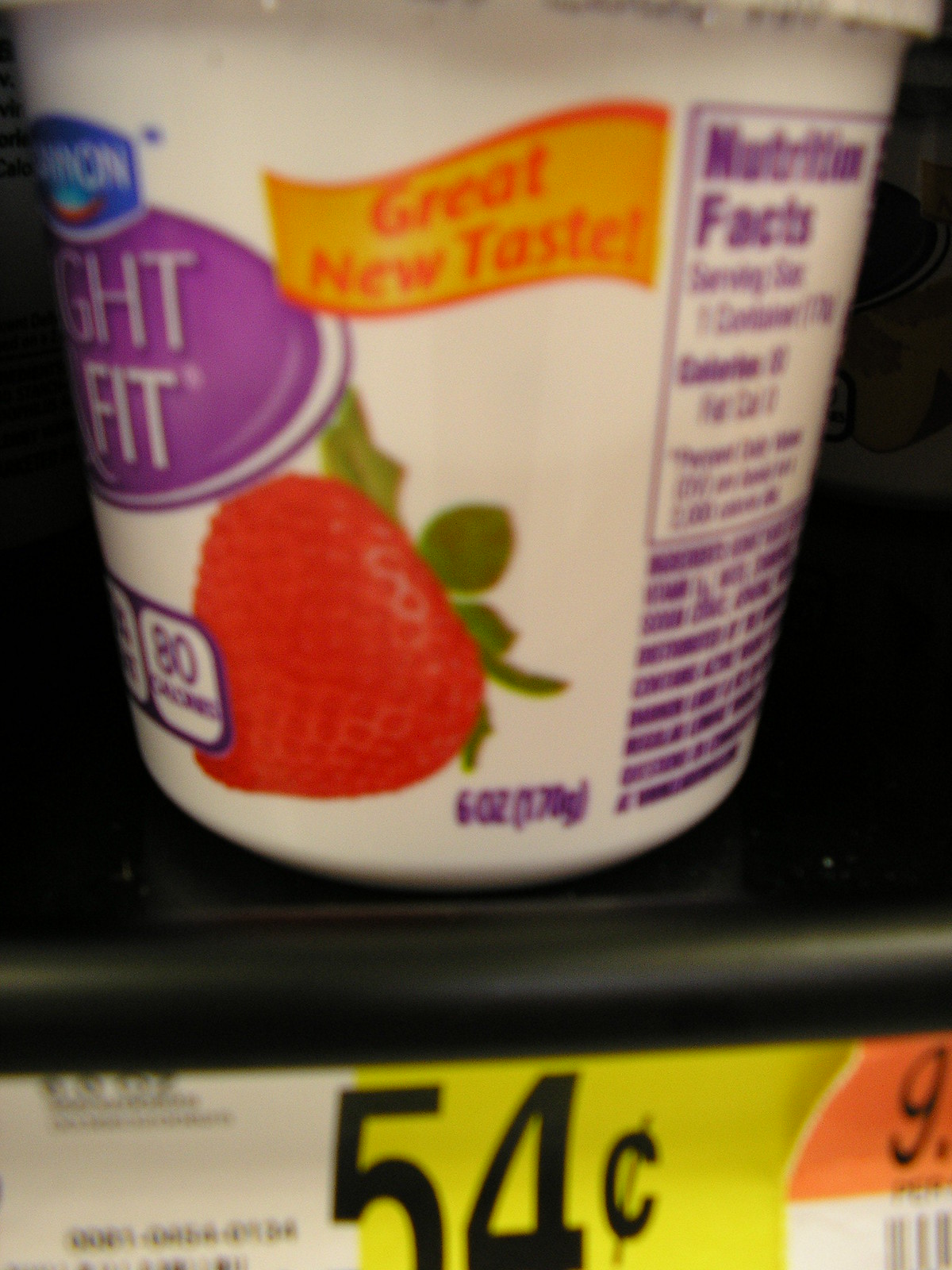In this blurry and low-resolution image, a circular white tub is prominently featured. The tub showcases an illustration of a vibrant red strawberry with green leaves. Beneath the tub, a price label can be discerned, though the exact details are unclear due to the image's quality. The tub is clearly labeled with "6 OZ (170 G)" indicating its weight.